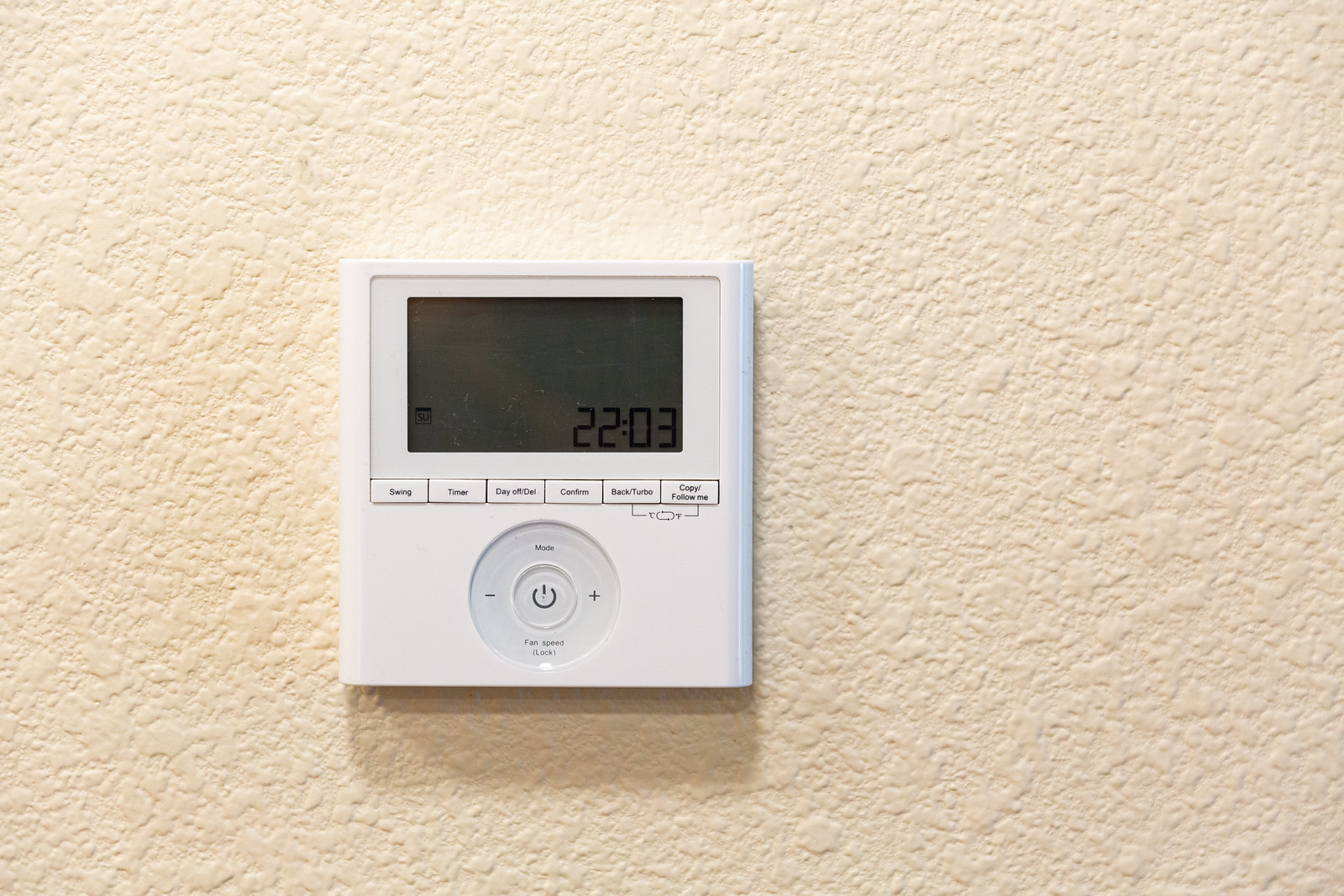The image depicts a wall-mounted thermostat set against a bumpy, textured, off-white background. The thermostat is positioned in the middle to the lower left-hand corner of the image. It features a gray digital display with black lettering, showing the time "2203" in military format, equivalent to 10:03 PM. Adjacent to the digital reading, there is a small square, and beneath this display, six rectangular white buttons are visible, although their labels are indistinguishable.

Beneath these buttons, there is a circular control panel with a prominent power button in the center, marked by the characteristic power symbol—a half-circle with a line at the top. To the left and right of this power button are minus and plus signs, respectively, indicating controls for adjusting settings such as temperature. While there are inscriptions at the top and bottom of the circular control panel, the text is not legible.